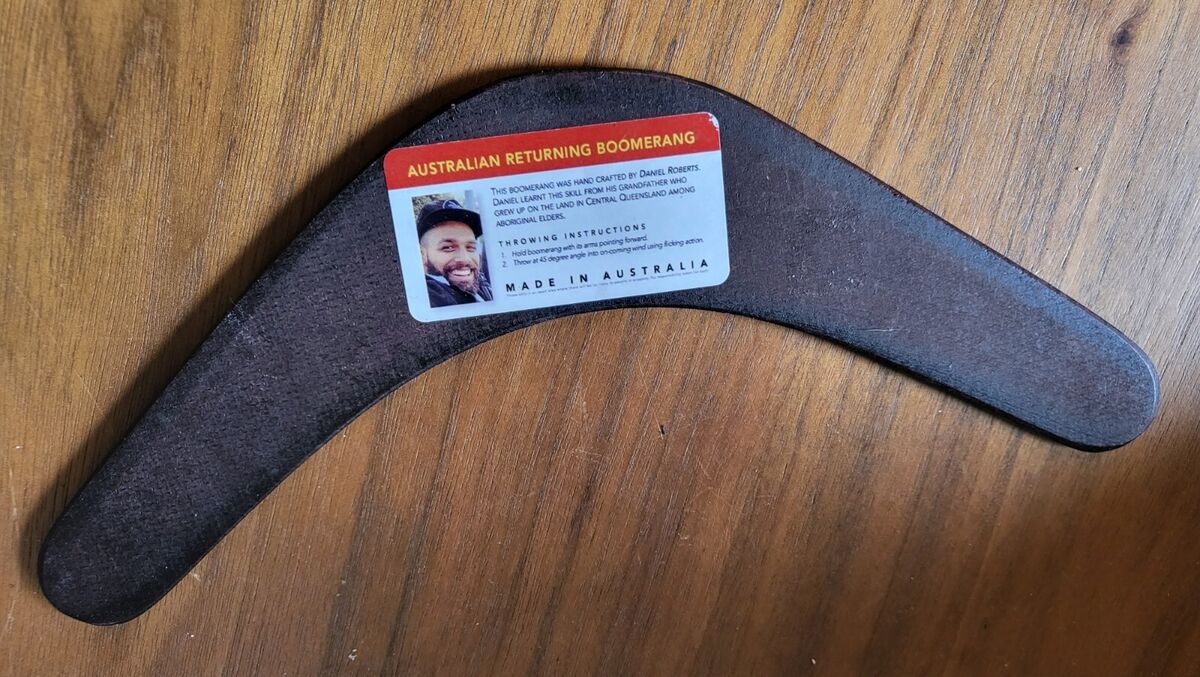This overhead color photograph captures a black boomerang positioned with its pointy part facing upwards, resting on a light brown wooden table marked with dark brown grains. The boomerang, though somewhat scuffed, features a smooth surface and rounded edges. A prominent label adorns the middle of the boomerang—its top border is red, and the main section of the label is blue with yellow text that reads "Australian Returning Boomerang." On the left of this label, there's a headshot of a smiling man wearing a black cap, identified as Danell Roberts, who learned the craft from his grandfather in central Queensland among aboriginal elders. The label also includes throwing instructions and the phrase "Made in Australia" in bold black letters at the bottom, with additional tiny text below. Notably, the wooden tabletop has a conspicuous cut in the middle, adding to the rustic setting of the photograph.